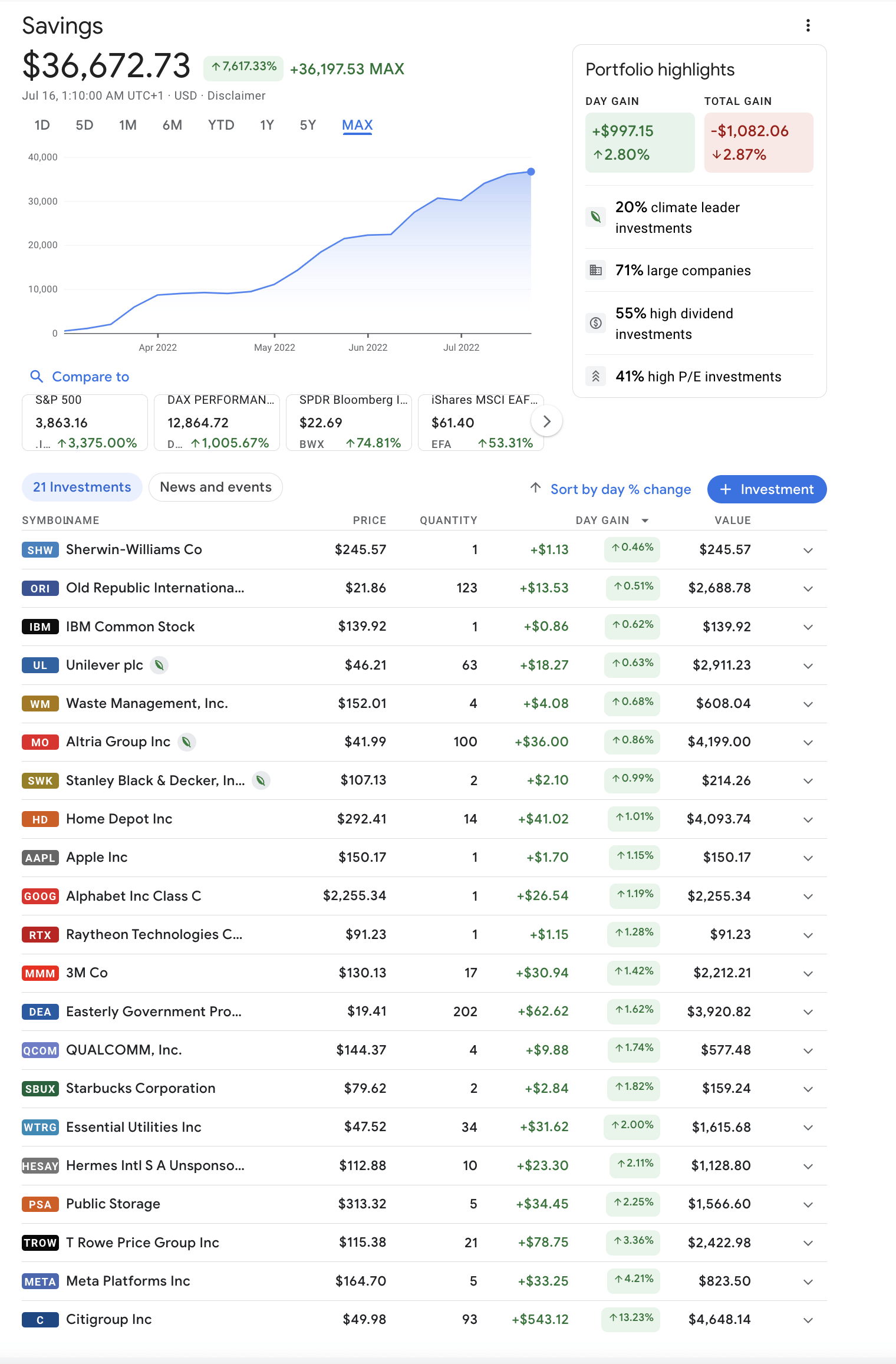A detailed image of a financial portfolio dashboard displayed on a white background. At the top of the page, the heading "Savings" is prominently shown with a balance of $36,672.73 and a percentage increase of 7.617%, which translates to a gain of $36,197.53. Directly beneath is the date, "July 16th". On the right side of this section, the "Portfolio Highlights" are displayed, showing both the "Day Gain" and the "Total Gain".

Below this section, on the left, is a blue graph illustrating the portfolio's performance trend over time. Beneath the graph, text indicates there are 21 investments in the portfolio. Adjacent to this is a "News and Events" tab. To the far right, features for sorting information by "Day Percentage Change" are provided. 

Additionally, a blue "Investment" button with white text and a white plus symbol is visible. Below this button, the names of various companies or brands are listed in a column. Accompanying each name, to the right, are columns indicating the "Price", "Quantity", "Day Gain", and "Value" for each associated investment.